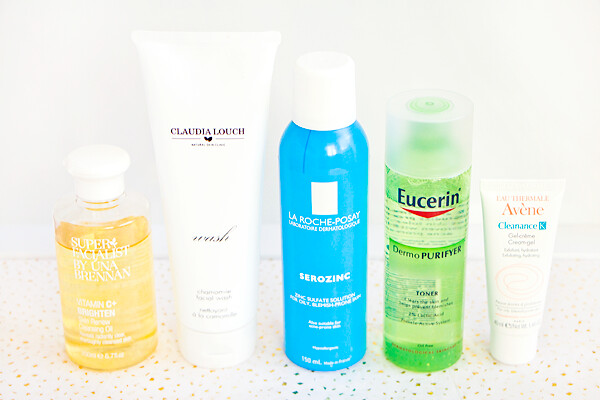This is a color photograph showcasing a collection of beauty products meticulously arranged on a white surface embellished with gold flecks. The backdrop consists of a plain white wall. Starting from the left, the first item is a nearly full, clear bottle with a white cap, labeled "Super Facialist by Una Brennan Vitamin C+ Brighten," containing a yellowish liquid. Next to it stands a sleek, tall white tube with the name "Claudia Louch" written in elegant purple letters, accompanied by a heart symbol, and a cursive "wash" on the front. Following this, there is a blue bottle with a white cap inscribed with "La Roche-Posay Laboratoire Dermatologique Serozinc." Adjacent to it is a green bottle labeled "Eucerin Dermo Purifier Toner" in black letters, topped with a frosted clear cap. Finally, on the far right, sits a small white tube marked "Eau Thermale Avène" with "Cleanance K" written in blue letters.